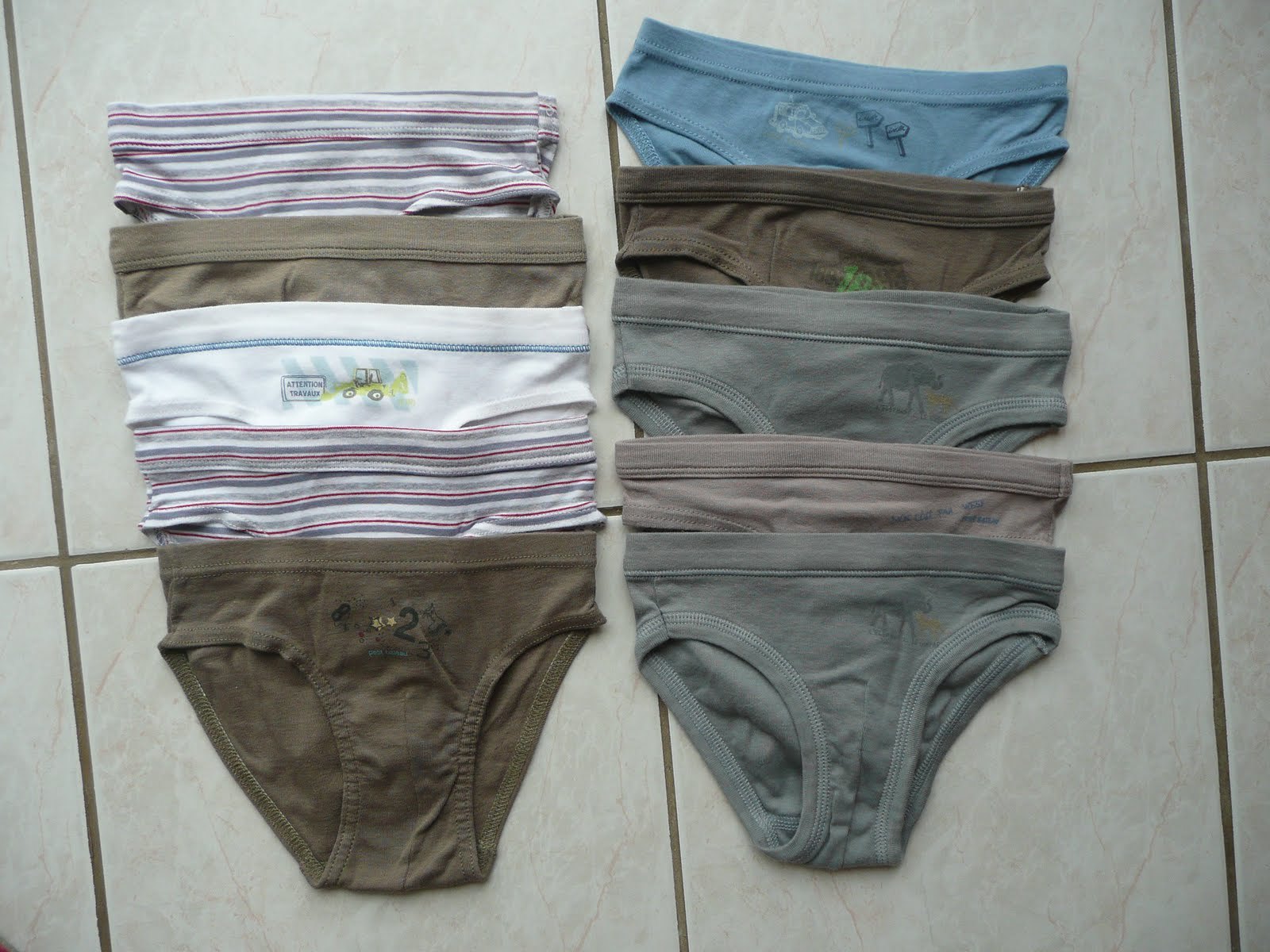This photograph, captured with an actual camera, showcases a meticulously arranged collection of children's underwear on a tiled floor. The floor features a greenish-gray coloration with dark grout lines, reminiscent of bathroom tiles. The underwear is arranged in two vertical columns, each containing five pairs.

In the left column, from bottom to top, the first pair is olive brown. Above that is a pink, white, and gray striped pair. The third pair is white, adorned with a yellow tractor and the word "Attention." The fourth pair is identical to the second, featuring the same pink, white, and gray stripes. The topmost pair in this column is another olive brown.

In the right column, starting at the bottom, the first pair is a gray with a moose design. The second pair is a brownish mauve. The third pair is gray, matching the bottom pair. The fourth pair displays a light brown color with a number "2" in the middle. The topmost pair is light blue with a truck and signs graphic.

The layout and repetitive design patterns suggest they might be part of an advertisement or sale display, highlighting a variety of designs in children’s high-crop underwear.